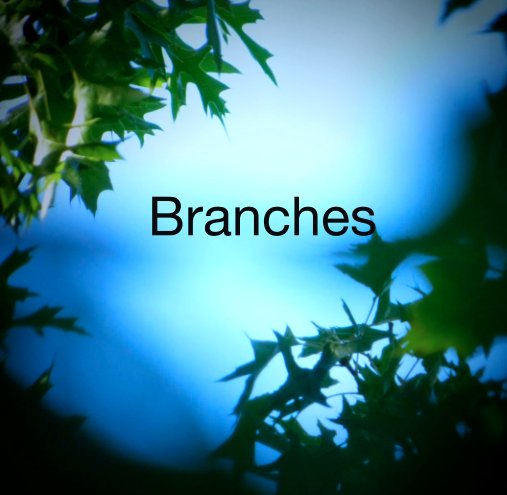The image depicts a serene scene resembling a nature photograph with a gradient background transitioning from light blue to dark blue, evoking a sense of dawn or twilight. The main focus is the text "branches" written in black ink, centrally positioned against the smooth blue backdrop. Green, sharp leaves frame the composition, concentrated heavily in the upper left and bottom right corners, resembling the view of looking up through tree branches. The blend of colors includes shades of blue, green, white, and black, contributing to the tranquil and slightly abstract aesthetic. This image could serve well as a visually pleasing slide in a PowerPoint presentation.